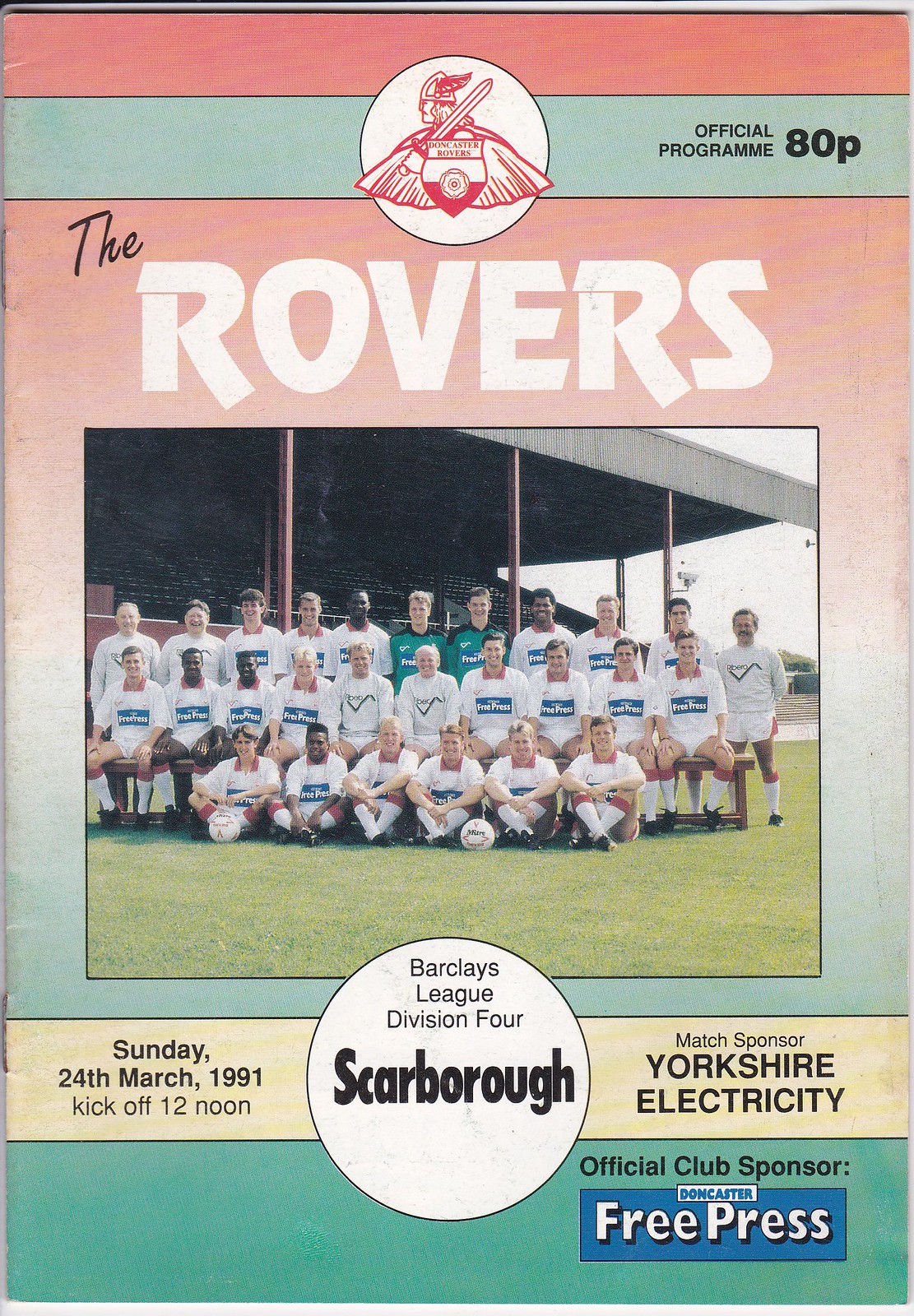In the image, an official program for the Rovers is prominently displayed. The title, "Program for the Rovers," is written in bold white font across the middle. Just beneath this title, a photograph captures the Rovers' team, all dressed in white uniforms. In the foreground, several team members are seated, holding soccer balls with their hands neatly folded on their laps. The second row features individuals sitting on chairs, while the third row has players standing.

Notably, two people among them are dressed in green uniforms. At the top of the program, the words "Official Program ADP" are inscribed, accompanied by an undecipherable red symbol enclosed in a circle. Further down, the program specifies the date and time: "Sunday, 24th March 1991, Kickoff 12 Noon." Below this, a circle with the words "Barclays League Division Four" emphasizes the league information in a larger, black font. The name "Scarborough" is highlighted in the same sizable font.

To the right of the image, additional details identify the match sponsor as "Yorkshire Electricity" and the official club sponsor as "Free Press," though there's an indistinct word above "Free Press" that remains unreadable.